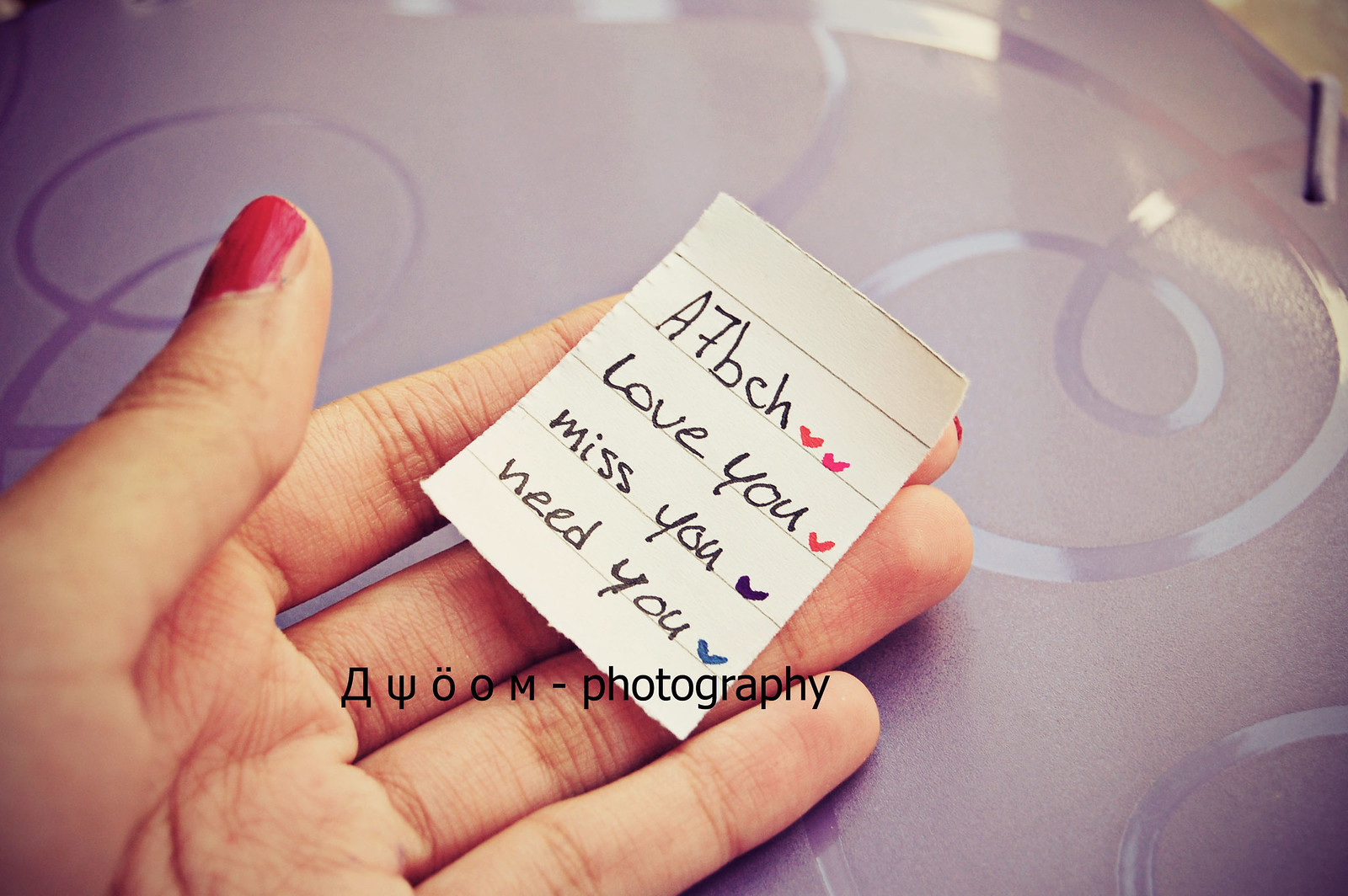A detailed close-up image of an older woman's hand, open-faced and adorned with reddish-pink nail polish, holding a small lined note. The note reads "A7BCH" followed by small red and pink hearts. Subsequent lines say "Love you" with a red heart, "Miss you" with a purple heart, and "Need you" with a blue heart. The hand rests on a purple surface with shiny purple swirls, and the upper right corner transitions to a yellowish background where the table drops off. Across the bottom of the note and the hand, the text "AYOOM-Photography" is visible in black ink, alongside some characters that appear to be in Russian or Greek.